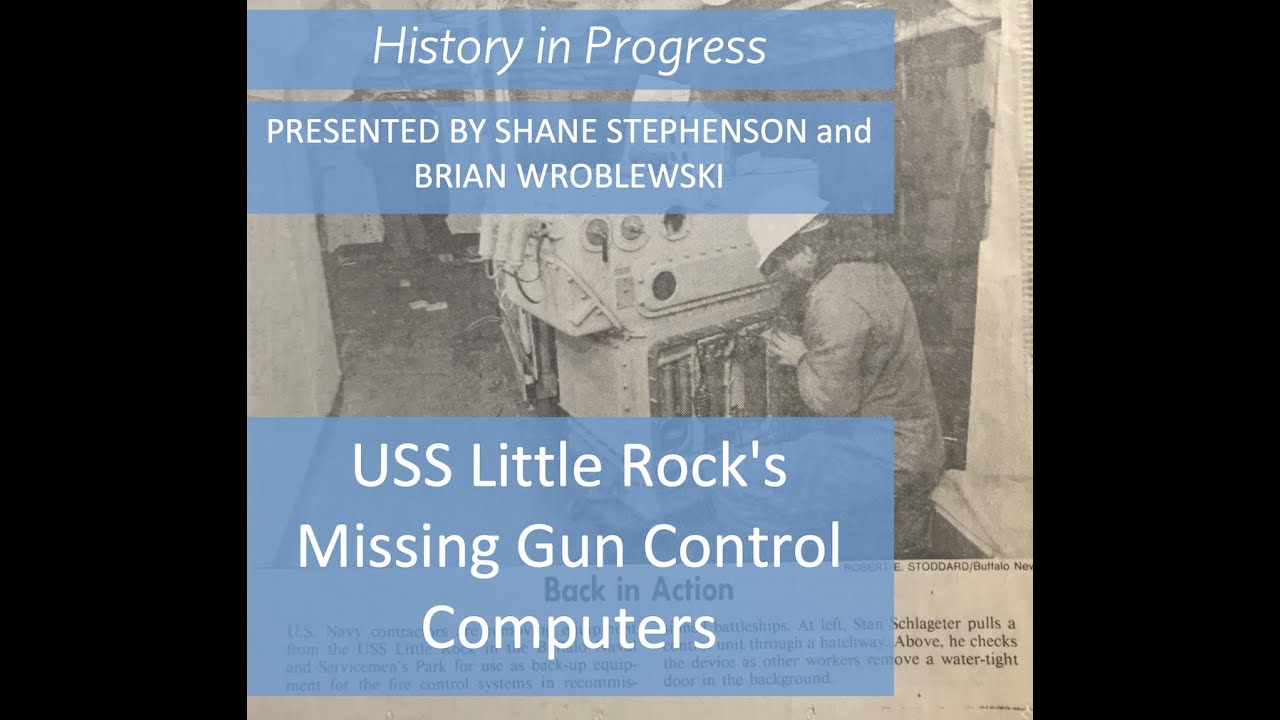The image features a clear, black and white newspaper clipping displaying a man with a white hard hat, crouched down and working on a large piece of machinery, likely an engine. The machinery, appearing cream-colored, is centrally located within the photograph, with black borders framing the image on the left and right. Overlaying this scene is text in white letters with blue backgrounds: "History and Progress, presented by Shane Stevenson and Brian Wroblewski," followed by "USS Little Rock's Missing Gun Control Computers." Near the bottom of the newspaper clipping, within partly obscured text, a visible headline reads "Back in Action." The overall setting of the image is brightly lit, ensuring the details in both the machinery and the man's actions are clearly visible.